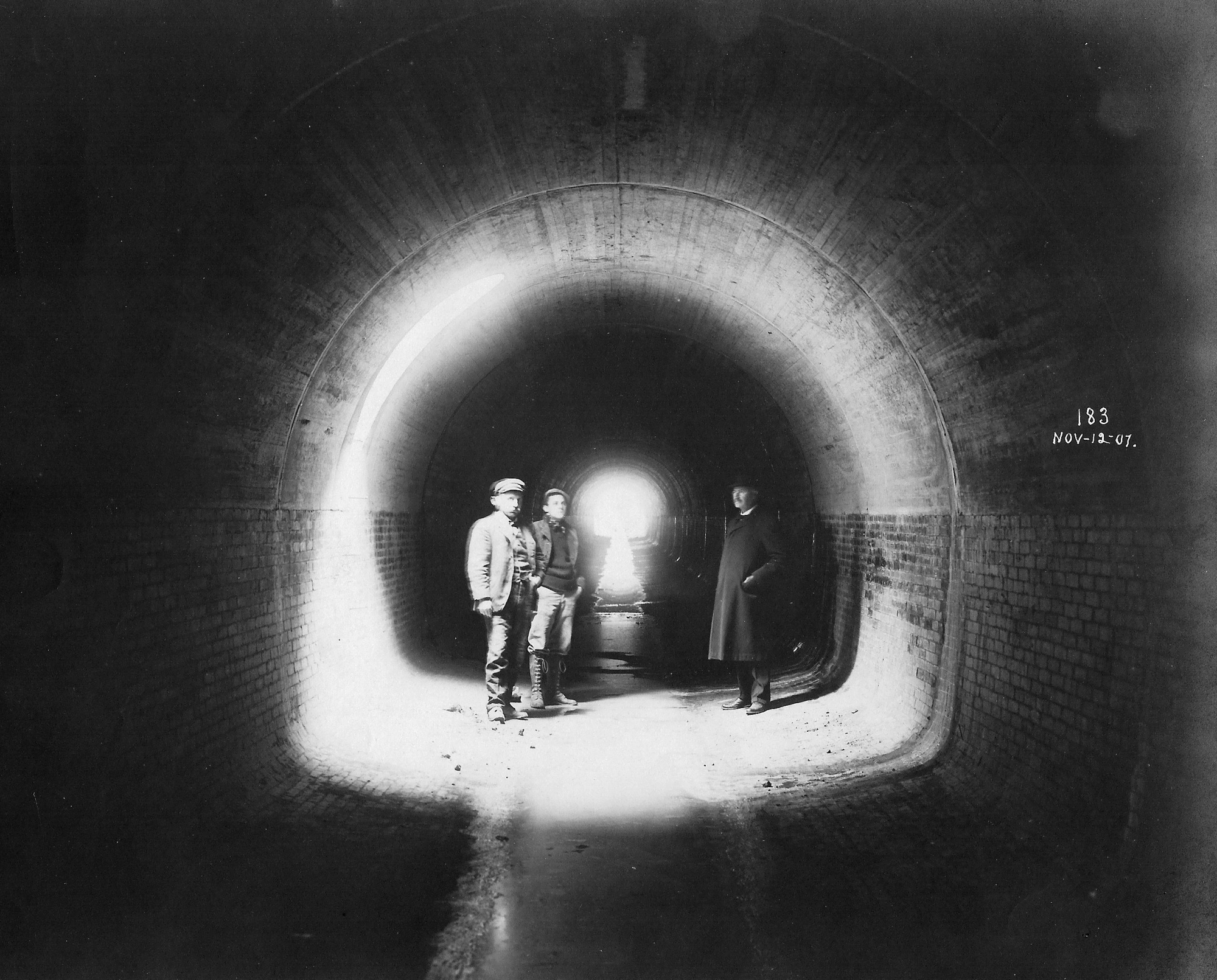The image is a rectangular black and white photograph from November 12, 1907. It has the number "183" written on the right-hand side. The scene depicts three men standing in an underground tunnel. The tunnel has brick walls that transition to a different material forming an archway at the top. The men are illuminated, with light casting shadows in the otherwise dark surroundings. The center of the tunnel, where they stand, is lit, and there is also light at the far end, suggesting an exit. 

On the right side of the image stands a man in a dark woolen overcoat and hat, with his hands in his pockets and wearing dress shoes. To the left, two men dressed in worker attire—shorter jackets, hats, and mustaches—stand side by side. One of the workers is notable for his tall lace-up boots and knickers. The quality of the photograph is poor, and shadows are cast by the lighting within the tunnel, which creates a dramatic contrast between the illuminated men and the surrounding darkness.